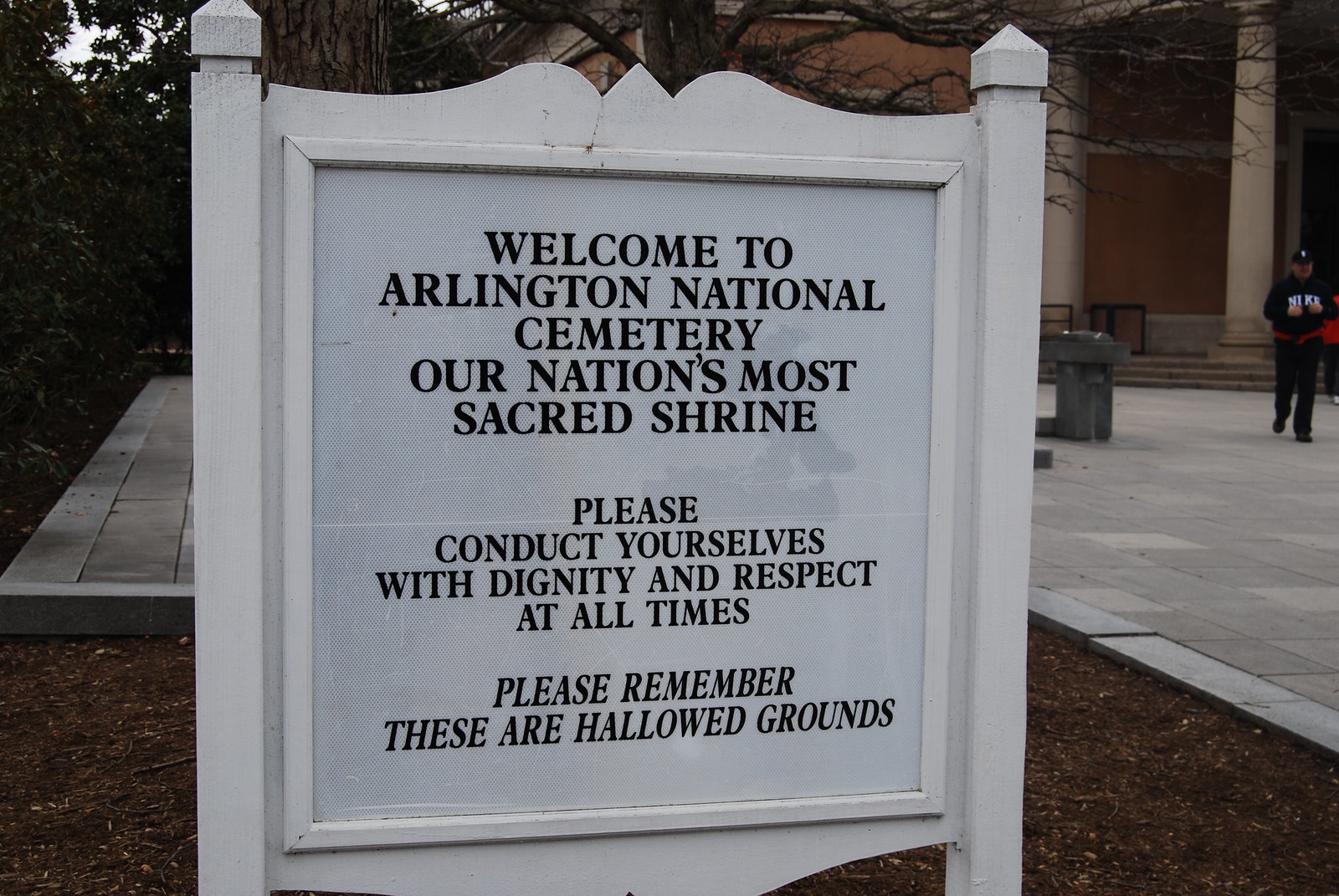The photograph features a close-up of a white wooden sign with black text, prominently displaying the message: "Welcome to Arlington National Cemetery, our nation's most sacred shrine. Please conduct yourselves with dignity and respect at all times. Please remember these are hallowed grounds." The sign is situated in a mulched area to the left of a concrete walkway. Behind the sign, a leafless tree extends its branches, indicating a winter setting. Partially visible in the background is a building with white columns. On the far-right edge of the image, a light-skinned male dressed in a black or dark blue sweatshirt, black pants, a jacket, hat, and possibly a baseball cap, walks along the concrete walkway. This composition emphasizes the solemnity and reverence associated with Arlington National Cemetery.